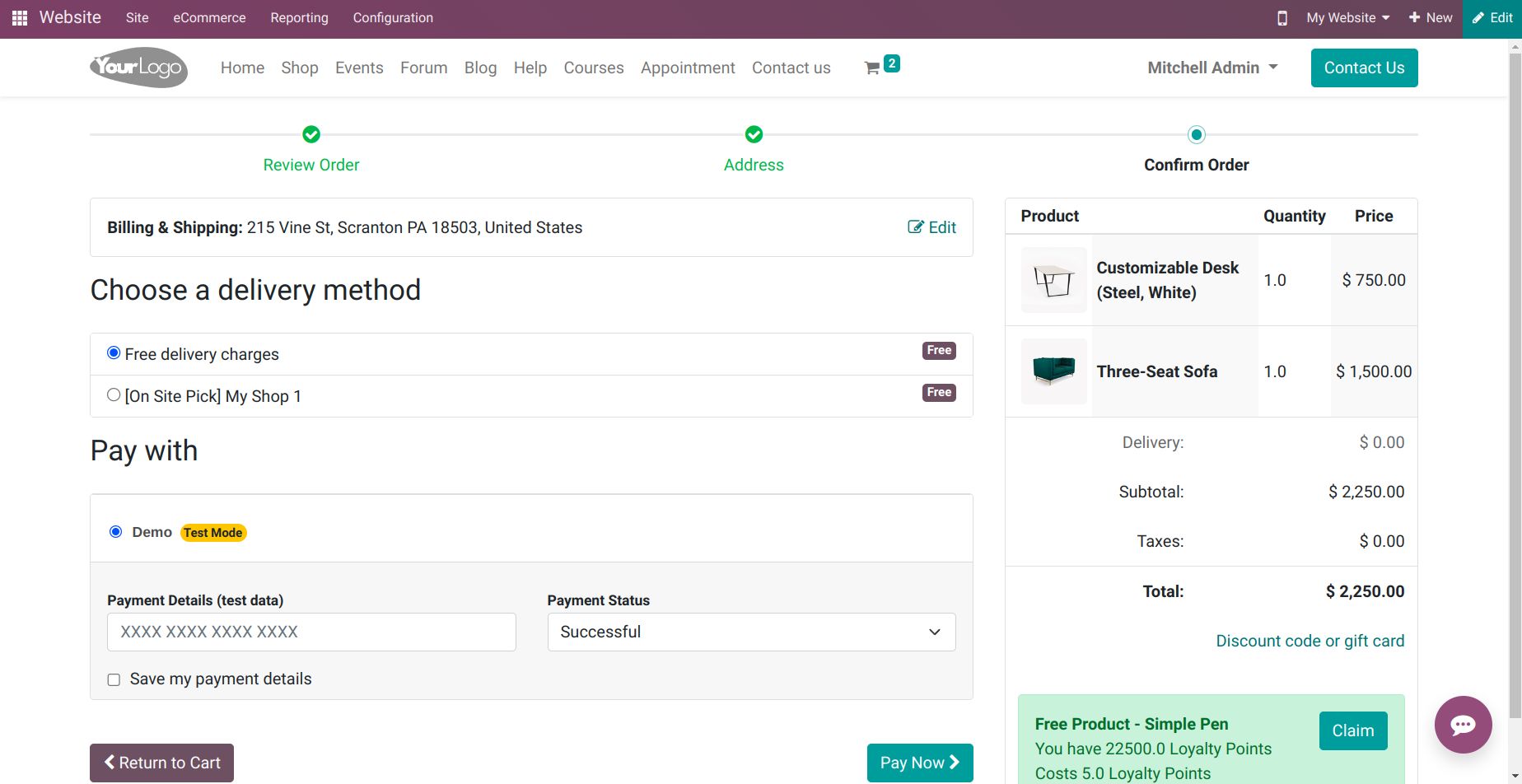The image depicts a detailed screenshot of a web page, showcasing its intricate layout and design elements. At the top, a header with a dark plum background features white text displaying "Website Site Ecommerce Reporting Configuration." In the upper right corner, "My Website" along with a pull-down arrow is visible, accompanied by a green "Edit" button featuring a pencil icon.

Directly below the header, the page is primarily white and houses an oval-shaped logo that reads "Your Logo." Adjacent to the logo is a horizontal navigation menu with links to "Home," "Shop," "Events," "Forum," "Blog," "Help," "Courses," and "Contact Us." To the right of the navigation menu sits an icon of a shopping cart with a green box containing the number "2." Furthermore, there is a green "Contact Us" action button beside it.

In the lower right corner of the page, there is a green box with dark green text that reads "Free Product: Simple Pen." A green "Claim" action button is positioned to the right of this text.